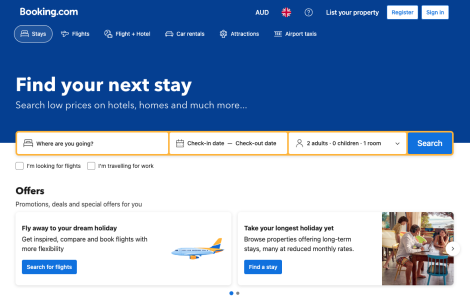The image showcases the UK version of the Booking.com website. The presence of a UK flag in the top banner confirms this. In the upper right corner, there are two buttons for user interactions: 'Register' and 'Sign-in'. 

Beneath these, a series of navigational tabs allows users to explore various services: 'Stays', 'Flights', 'Flight + Hotel', 'Car Rentals', 'Attractions', and 'Airport Taxis'. A promotional text reads, "Find your next stay, search low prices on hotels, homes, and much more."

A user input section consists of multiple entry fields where users can specify their travel details. They can type their destination city, select check-in and check-out dates, specify the number of adults, and choose the number of rooms required. To the right of this section, a prominent blue 'Search' button allows users to execute their searches.

Below this search section, there are checkboxes labeled 'I’m looking for flights' and 'I’m traveling for work', offering additional customization options. At the bottom of the page, special offers and promotions are displayed, including enticing messages such as "Fly away to your dream holiday," "Search for flights," and "Take your longest holiday yet, find a stay."